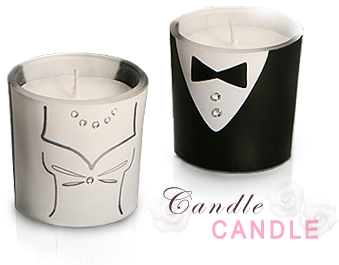This color photograph, in landscape orientation, showcases a pair of cylindrical white candles set in silver liners, with intricately designed holders that symbolize a bride and groom. The candle on the left has a woman's wedding dress design, featuring a scooped neckline adorned with a beaded necklace, white satin bodice, and details down to the waist, creating the look of a bridal gown. The candle on the right represents a man's tuxedo; this design includes a black bow tie, black jacket, white shirt with two rhinestone buttons, and an inverted white triangle mimicking an open shirt. Both candles have small white wicks protruding from the center. Set against a stark white background that creates a reflective surface below, the bottom right corner of the image displays the word "CANDLE" twice: the first in a black script font and the second in all caps, light pink sans serif. This detailed imagery and text layout evoke a sense of wedding celebration, ideal as a gift for newlyweds.